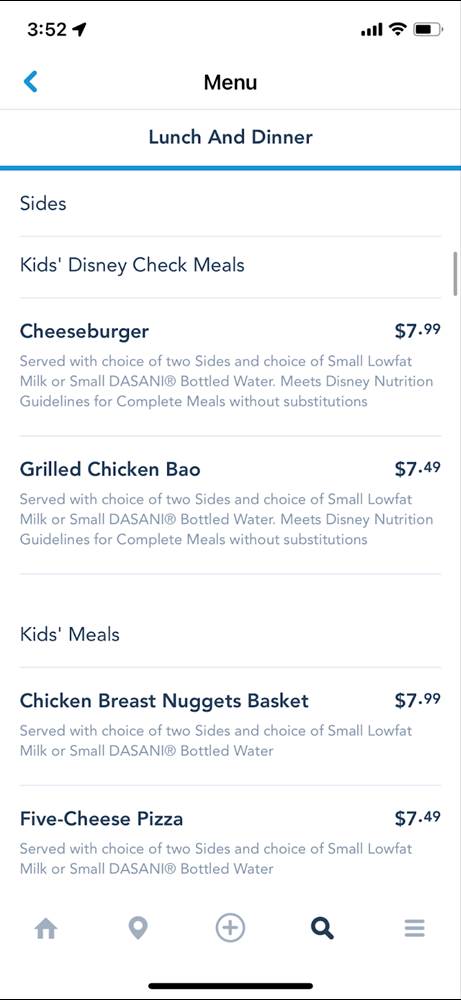This is a screenshot taken from a mobile phone, featuring a predominantly white background. At the top of the screen, various phone status icons and information are visible in black font. The time is displayed as 3:52. Location sharing is enabled, the Wi-Fi and mobile signal indicators are full, and the battery level is at 75%.

Below the status bar, the following text details a menu:

- The first line says "Menu" in black font, followed by a horizontal black line.
- Underneath, it reads "Lunch and Dinner," followed by a blue line.
- Below this, it says "Sides," followed by another black line.
- The next section is labeled "Kids Disney Check Meals," again followed by a black line.

The menu items for kids include:

1. Cheeseburger: 
   - Description: Served with a choice of two sides and a choice of small low-fat milk or small Dasani bottled water.
   - Note: Meets Disney nutrition guidelines for complete meals without substitutions.
   - Price: $7.99

2. Grilled Chicken Bao:
   - Description: Served with a choice of two sides and a choice of small low-fat milk or small Dasani bottled water.
   - Note: Meets Disney nutrition guidelines for complete meals without substitutions.
   - Price: $7.49

3. Chicken Breast Nugget Basket:
   - Description: Served with a choice of two sides and a choice of small low-fat milk or small Dasani bottled water.
   - Price: $7.99

These items are organized under the section titled "Kid's Meals."